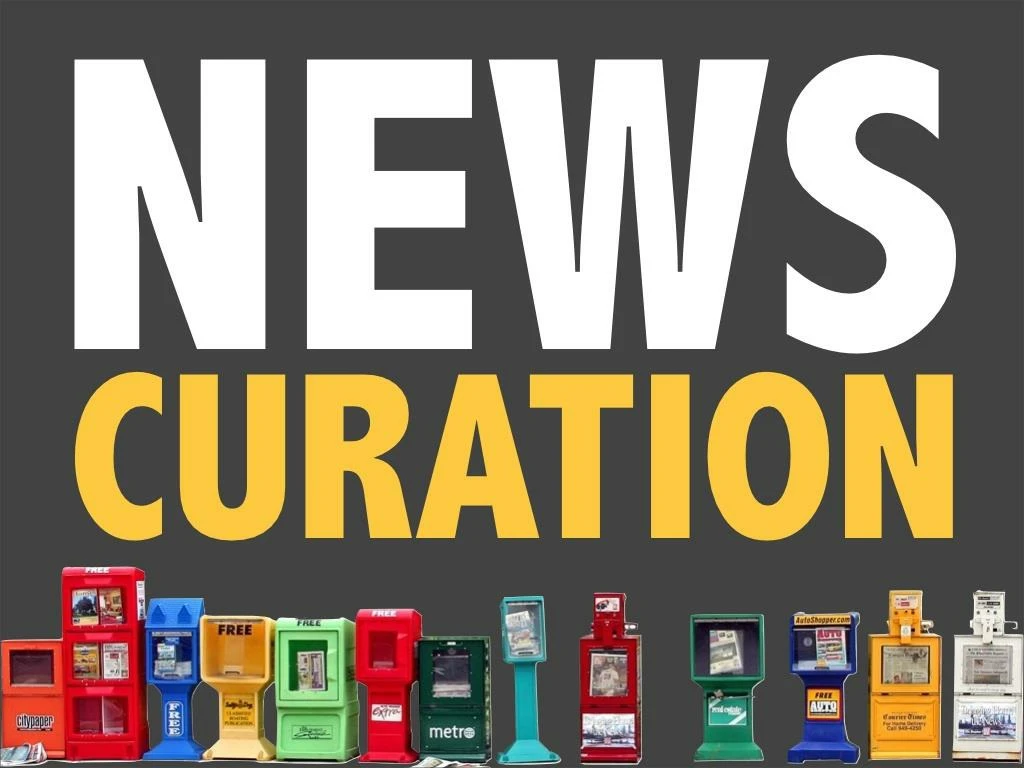The image features a dark green background with the text "NEWS CURATION" dominating the top two-thirds. "NEWS" is written in large, white, all-caps letters, taking up almost half the image, while "CURATION" appears in a slightly smaller, two-thirds size, in bright yellow all-caps letters below it. The bottom third of the image showcases a row of ten diverse newspaper vending machines, varying in colors such as red, blue, green, white, and yellow. These old-fashioned stands, which resemble those you might find on a city street, come in different varieties—some requiring coins to release the newspapers, with pull-down or pull-up handles, and others marked "FREE." All the vending machines are positioned to face the viewer directly, making their colors and designs clearly visible.